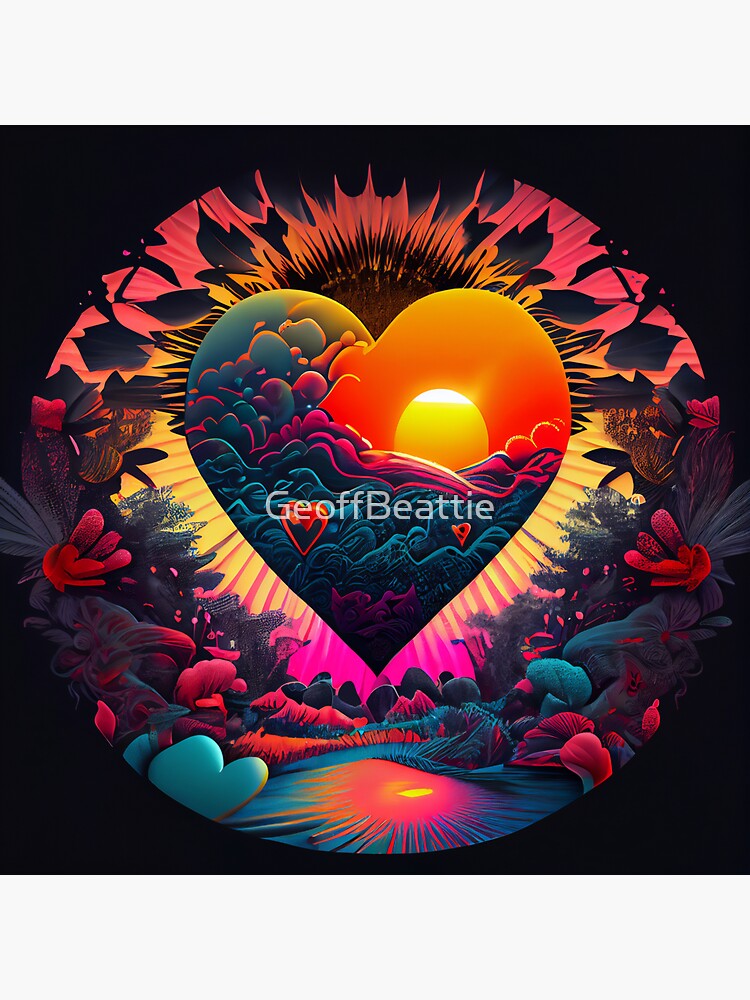This image is a vibrant and detailed piece of art, possibly a painting or computer-generated graphic. The backdrop is entirely black, adding depth and contrast to the scene. Central to the composition is a large heart that contains a striking visual narrative: the right side of the heart features a radiant sunrise with orange and yellow hues, while the left side appears to be underwater, casting an aqua tone. Surrounding this heart is a circular border filled with an array of multicolored flowers, including shades of pink, red, blue, and orange, creating a lush, forest-like effect that complements the heart. A serene lake also seems to be part of this encompassing scene. The heart and its encircling floral landscape are illuminated with yellow rays, which cast a yellow and pink shadow on the ground below. Prominently within the heart is the artist's signature, "Jeff Beattie," adding a personal touch to this intricate and harmonious artwork.